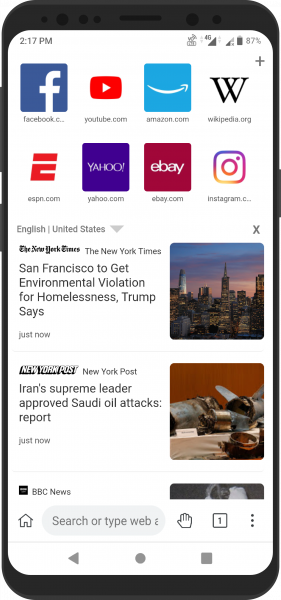In this detailed image, a mobile device displays a webpage with various app icons. The time on the device reads 2:17 PM. At the top left, the 4G icon and network signal bars for SIM1 and SIM2 are visible. On the right side, the battery percentage is shown at 87%. The webpage features app icons for several websites, including facebook.com, yahoo.com, youtube.com, amazon.com, geekpedia.org, espn.com, ebay.com, and instagram.com. Notably, a headline on the page reads, "San Francisco to get environmental violation for homelessness, Trump says."